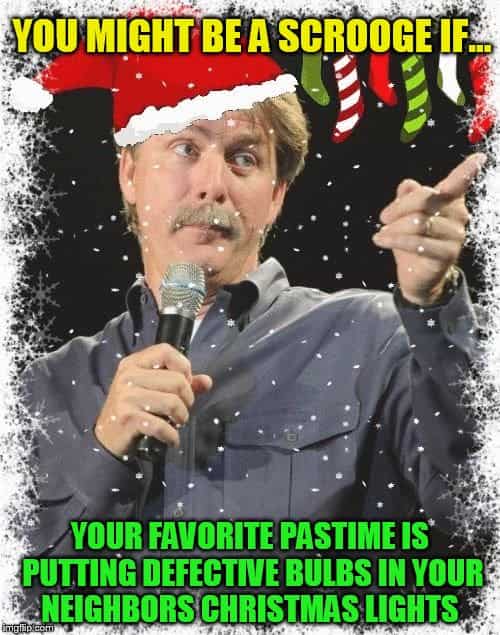The meme features a holiday-themed, digitally edited photograph of comedian Jeff Foxworthy. He is wearing a clip-art style Santa hat with red fabric and white trim, and his right hand is holding a black microphone close to his mouth. Foxworthy is looking to the right with a slight, smug expression as he points his left finger outward, reminiscent of his famous "you might be a redneck" jokes. He is dressed in a gray button-up shirt with a collar and two chest pockets, over a white undershirt.

The meme is bordered by illustrations of icicles and snowflakes on a black background, giving a frosty winter effect. At the top of the image, yellow text reads, "You might be a Scrooge if..." Below, in green text, it humorously concludes, "your favorite pastime is putting defective bulbs in your neighbor's Christmas lights." In the top right corner of the image, there’s a string of clip-art Christmas stockings in a sequence of colors and patterns: green, red and white stripes, solid red, green and dark green stripes, white with dark green accents, and another solid red. The overall design combines elements of festive graphics and Jeff Foxworthy’s comedic style to create a humorous holiday meme suitable for social media sharing.